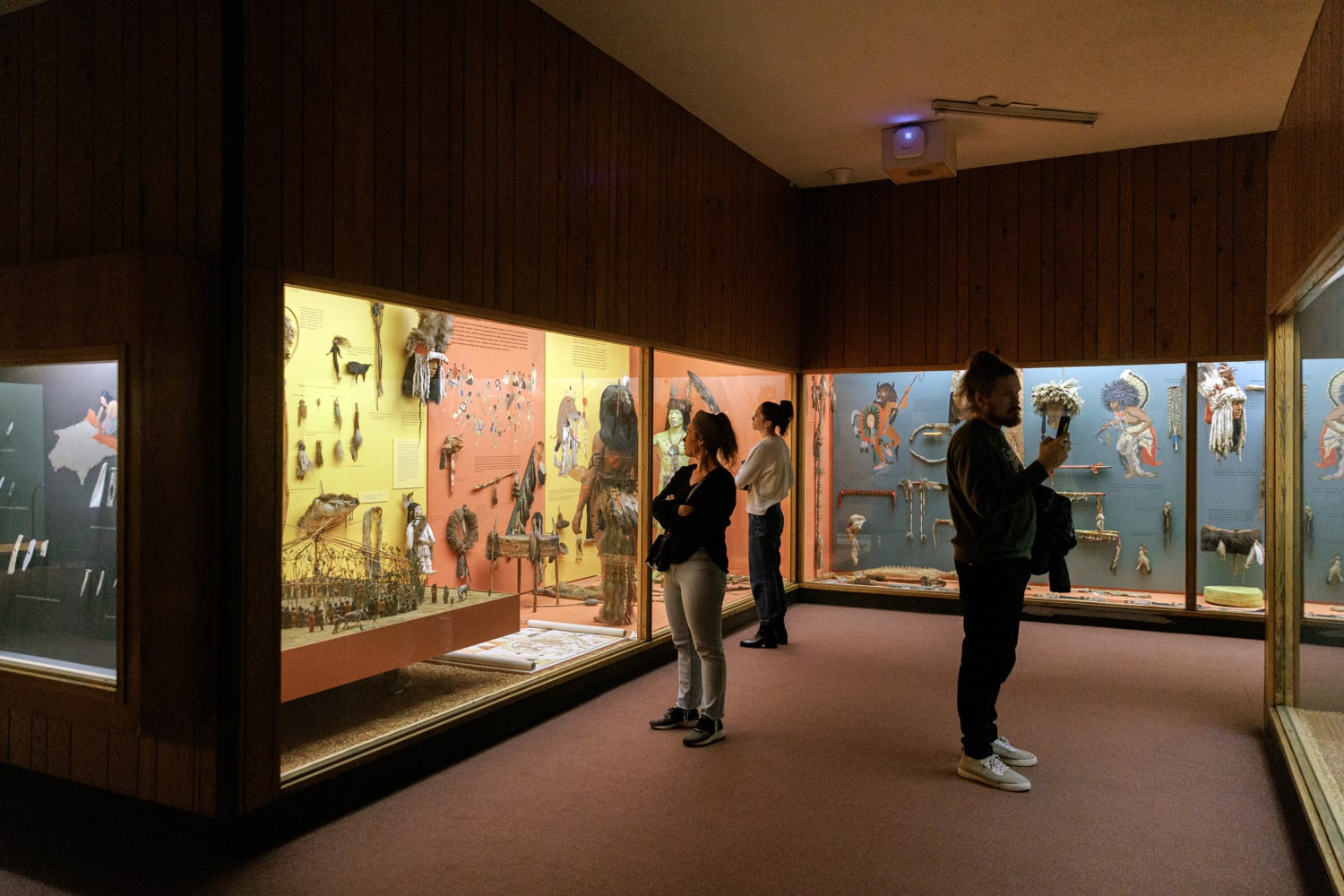In this vividly detailed photograph taken inside a museum, the scene is dominated by a long display case showcasing indigenous artifacts, such as tools, headdresses, and weapons. The ceiling is white, featuring a camera or monitor, while wood paneling adorns the area above the display cases. The display cases are tall, with glass nearly reaching the terracotta-colored floor, allowing viewers to see the contents clearly. 

Three people are examining the displays intently. On the left, two women stand with arms crossed, each engrossed in a different section of the case. The woman furthest back wears a white top and dark pants, while the closer woman has a black top paired with lighter-colored pants and a purse over her shoulder. On the right, a man with a top bun and beard, dressed in sweats and white sneakers, is capturing a photo with his phone. 

In the display cases, alongside the indigenous artifacts, arrows, and feathers are visible under varying colored backgrounds—one blue and another yellow and red. The detailed setup and diverse apparel of the viewers create a scene rich in cultural exploration and human curiosity.